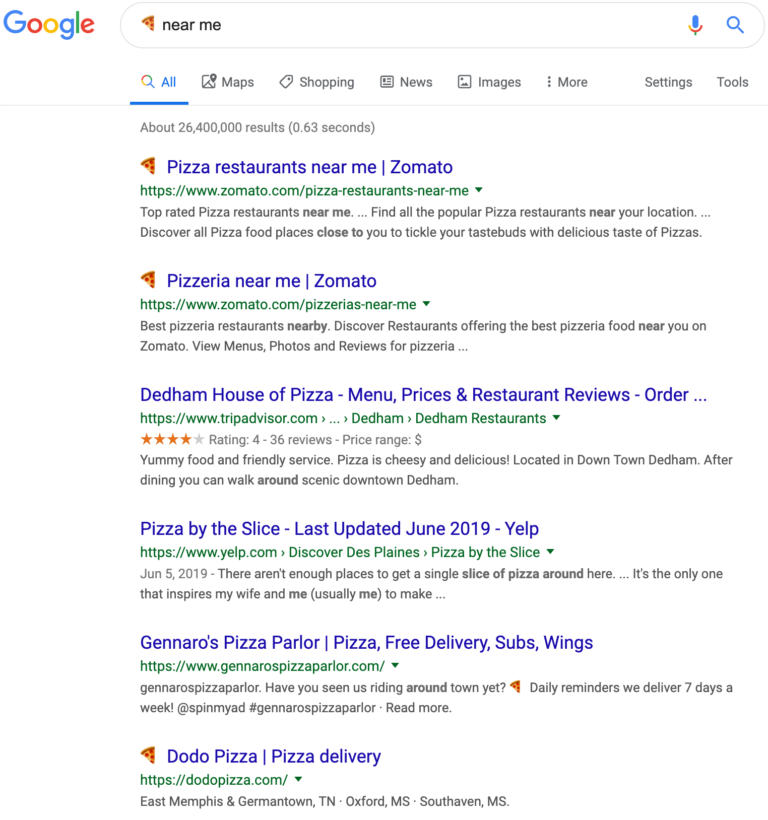This image is a detailed screenshot of Google search results for the query "pizza near me." The iconic Google logo is prominently displayed in the upper left corner, adjacent to the capsule-shaped search bar. Within this search field, there's an emoji of a pizza slice followed by the text "near me." 

On the far right of the search bar, the classic Google microphone icon and magnifying glass symbol are visible. Beneath the search bar, the menu options include "All," "Maps," "Shopping," "News," "Images," "More," "Settings," and "Tools," with "All" currently selected. 

Directly below these options, it notes that there are approximately 26,400,000 results, retrieved in 0.63 seconds. The visible portion of the search results shows six entries, three of which are marked with a small pizza emoji to their left.

Each search result is formatted with a blue or purplish clickable title, a green URL beneath it, and gray descriptive text. Some entries also include ratings. The top result is "Pizza restaurants near me - Zomato," followed by "Pizzeria near me - Zomato." The third result is "Dead Ham House of Pizza - Menu prices and restaurant reviews, order..." which includes four stars from 36 reviews. Subsequent entries are "Pizza by the Slice - Yelp, last updated June 2019," "Gennaro's Pizza Parlor - Pizza, free pickup, delivery, subs, wings," and the final result, "Dota Pizza - Pizza delivery."

This search results page provides a variety of local pizza establishments with various services, star ratings, and review counts, catering to the user's query for nearby pizza options.